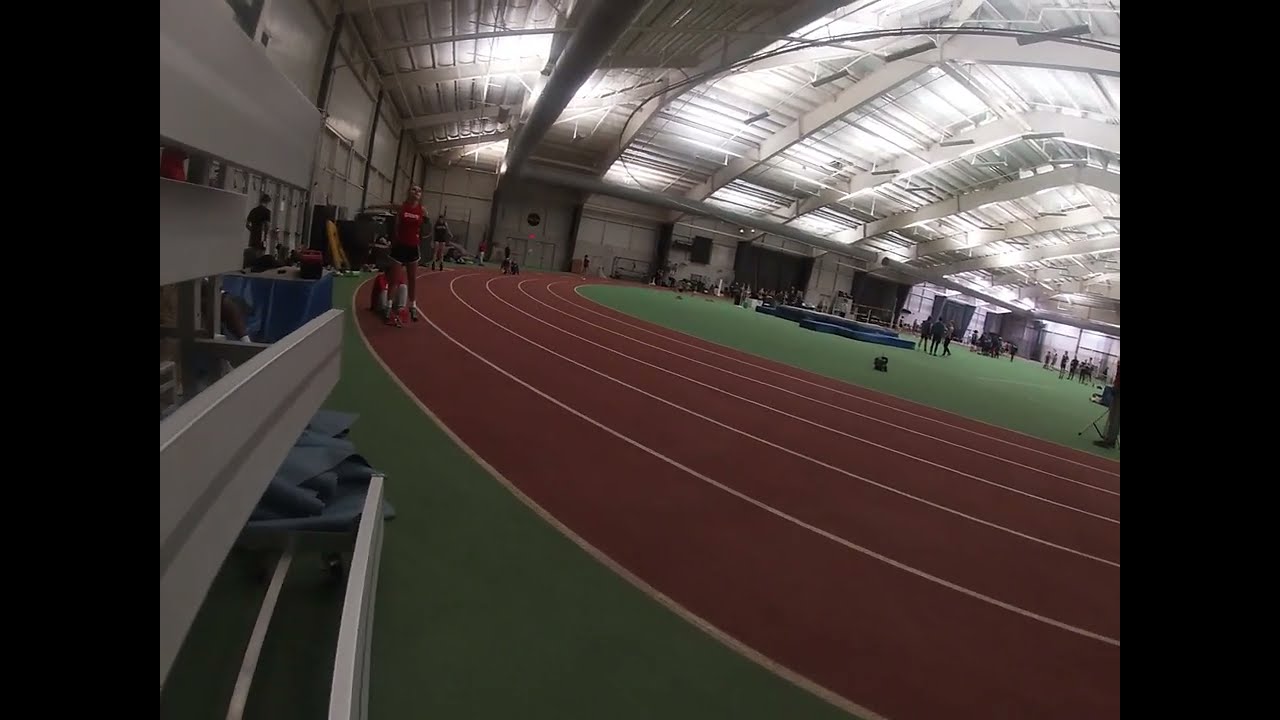The photograph showcases an indoor track and field facility, characterized by its bright lights and high, metallic ceiling with triangular support beams. The central area consists of a green artificial grass surface, surrounded by a circular track with six lanes marked by white lines on a brownish-red surface. The interior walls appear gray and metallic. Prominently featured is a woman in a red shirt and black shorts standing on one of the tracks. Another person in similar attire can be seen sitting nearby. Additional figures, blurred and less distinct, can be observed both near the bench and milling around the center green area—likely athletes preparing for events. The image is taken at an angle and lacks professional polish, capturing the dynamic atmosphere of the indoor athletic facility. Colored details within the scene include black, white, gray, silver, red, green, tan, brown, and blue elements.